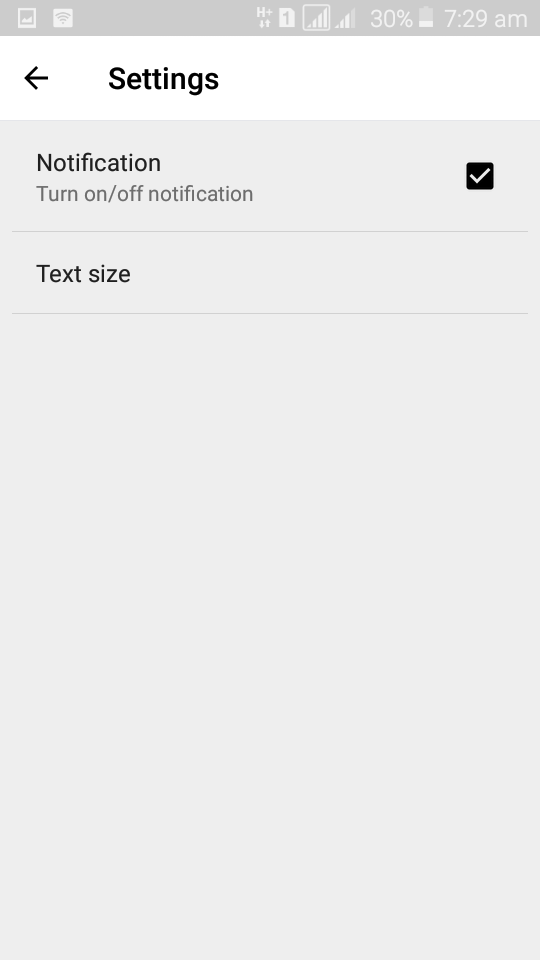This image is a cropped screenshot of a cellphone's settings panel. At the top, there is a white banner that spans the width of the screen. In this banner, the word "Settings" appears in bold black letters at the top left, with an arrow pointing to the left just before it. The portion to the left of "Settings" is blank.

Below this banner, the background of the screenshot transitions to grey. On the top left, directly under the white banner, is the heading "Notifications" in bold black font. Beneath this heading, there is a subtext that reads "Turn on/off notifications." To the right of this text, there is a checkbox that is currently checked, indicating that notifications are enabled.

Further down, there is another setting labeled "Text Size" in smaller, bold black letters. The remainder of the panel is vacant grey space as the bottom part of the screen is cut off, making the home buttons or any other interface elements invisible.

At the very top of the screenshot, a darker grey status bar displays several icons including the telephone, the current time, the battery icon with its percentage, the Wi-Fi signal strength, and the cellular signal strength icon.